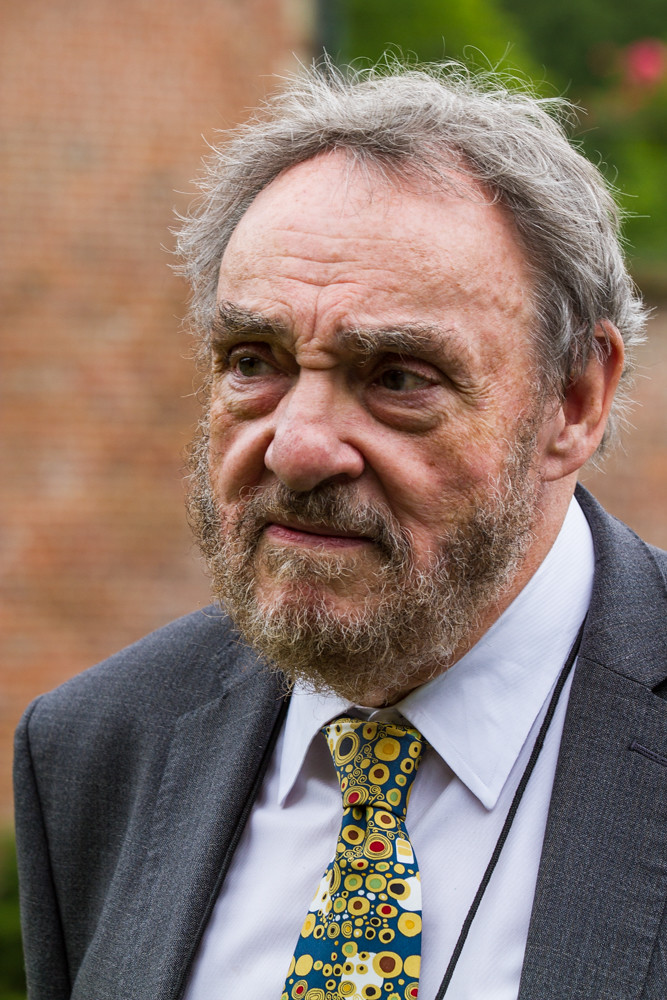The image captures a close-up of a man, identified as British actor John Rhys-Davies. He possesses short, scraggly gray hair with bald spots, a bushy gray and brown beard, and thick eyebrows. John is shown standing at an angle, looking off to his right, as if listening to someone speak. He wears a light blue shirt accompanied by a dark blue tie adorned with a pattern of golden circles and multicolored centers—red, green, and blue among them. He also has on a gray wool suit jacket that's open, revealing his shirt and tie. An attentive, serious expression is etched on his face. The background is blurred, featuring colors of brown, light brown, green, and hints of pink, suggestive of a brick wall and some greenery with flowers.